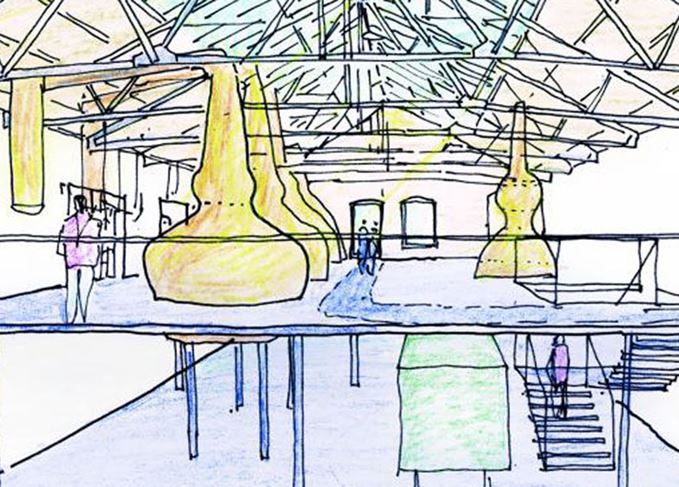The image is a colored drawing depicting the interior of a factory. The factory has two levels, with visible structural supports such as pillars and exposed ceiling rafters. The drawing features a series of four yellow objects that resemble pieces from the game Sari or oil cans. There is a distinct pathway that starts at a door in the background and leads to the foreground, continuing down a set of stairs to the bottom level. 

On the lower level, there's a green rectangular machine and the blue floor. The scene includes several figures: one person in a pink shirt is descending the stairs, another person in pink is standing near the rail on the top level, and two other figures in blue attire are on the pathway. The composition captures various construction elements and machinery within this industrial setting.